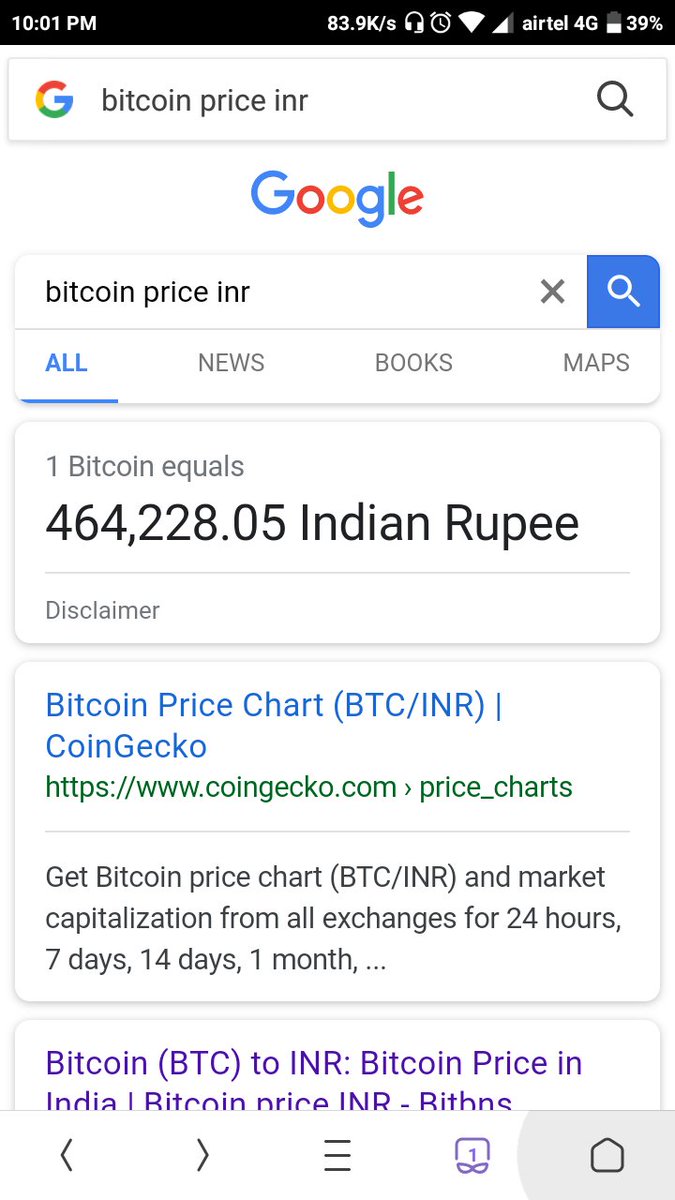A detailed screenshot of a cell phone screen is captured, featuring various elements. At the top, a black status bar displays key information: the current time is 10:01 p.m., and an ongoing data transfer rate is 83.9 kilobytes per second. This is followed by several icons indicating different statuses — a headphone icon, an alarm icon, a Wi-Fi connectivity symbol represented by a pizza slice, and a signal strength triangle showing three out of four bars. Additionally, it shows the network provider as Airtel 4G. The battery icon reveals that it is less than half full, and the accompanying text indicates it is at 39%.

Below this status bar is a search bar adorned with the Google "G" logo on the left and a magnifying glass icon on the right. The text within the search bar reads "Bitcoin price". The screen's content includes a search result header displaying "Google Bitcoin price INR" and tabs labeled "All", "News", "Books", and "Maps" with "All" being selected.

The top search result shows that one Bitcoin equals 464,228.05 Indian Rupees, accompanied by a gray disclaimer note beneath it. Another result appears below, titled "Bitcoin price chart BTC/INR" from iCoin Gecko, which offers a detailed view of the Bitcoin price chart and market capitalization, including time frames of 24 hours, 7 days, 14 days, and 1 month.